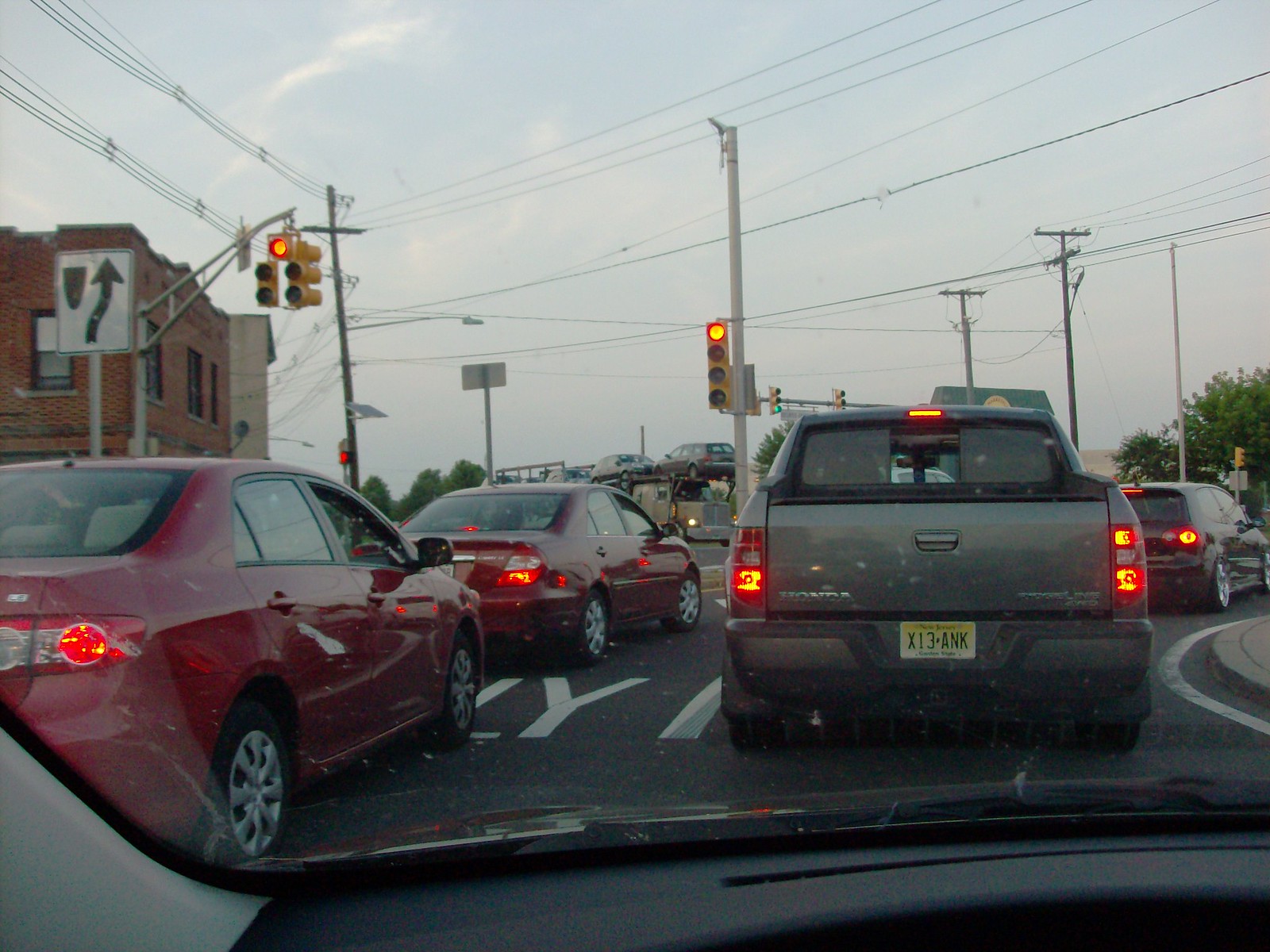The image captures a scene from inside a car, viewed from behind the driver’s seat, revealing the black dash ahead. The car appears to be stuck in a traffic jam, waiting at a red traffic light. Directly in front is a gray Honda Ridgeline with a yellow license plate reading X13ANK. To the left, in the adjacent lane, are two red sedans, with a brick building behind them. The sky is a light blue-gray with faint clouds visible. Down the road, there's a big semi-truck hauling cars on its top and bottom decks. Overhead, power lines on wooden posts crisscross through the scene. Trees are visible in the distance, indicating the setting is likely in a downtown area with the road curving ahead, suggesting possible directions to either left or right.